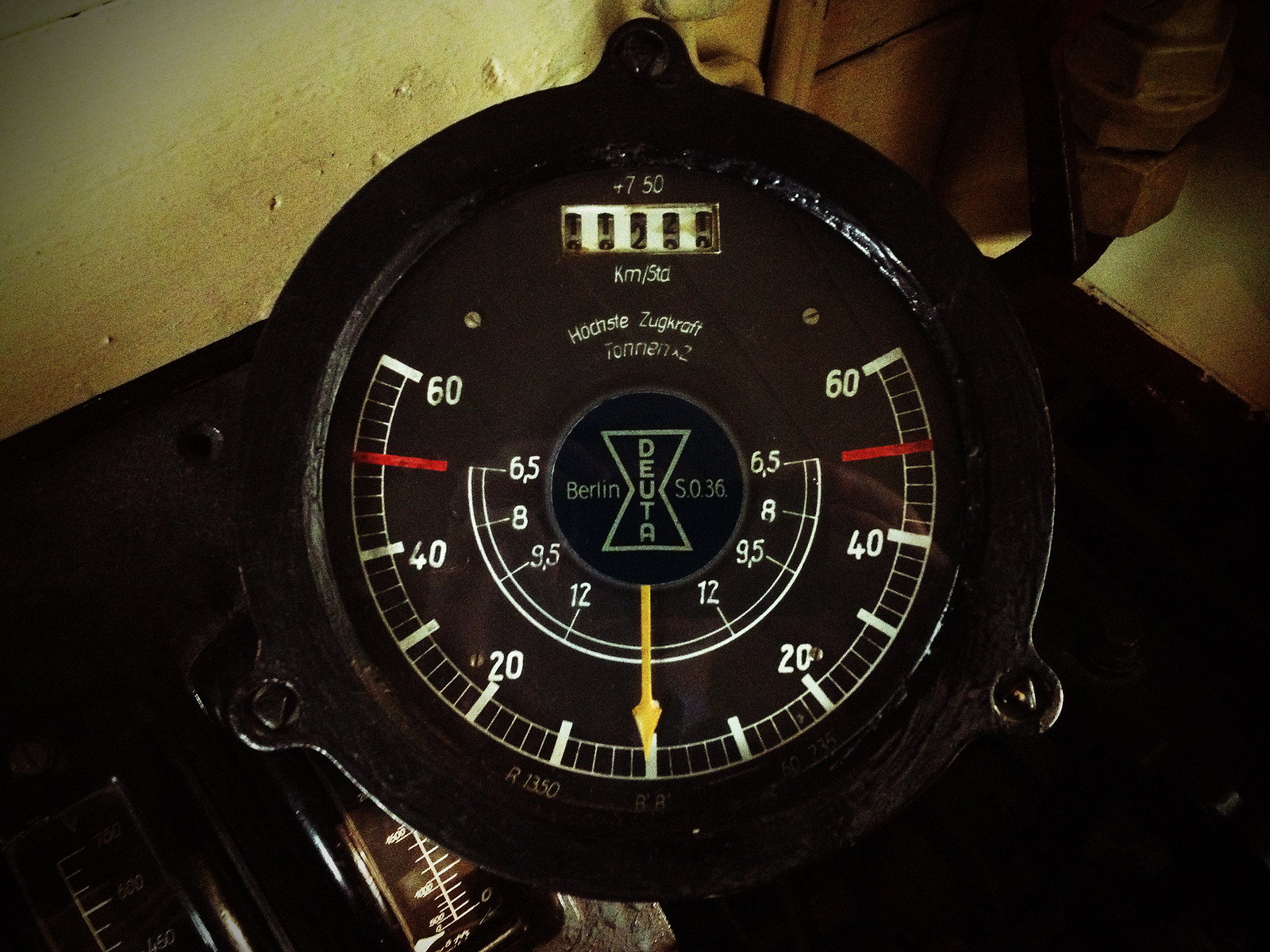This photograph, taken in a garage or workshop, prominently features a large black mechanical device in the center, set against a backdrop of a slightly dirty, poured concrete wall in the upper left corner. Below the wall is a broad black workstation surface occupying much of the lower section of the image.

The focal point is a circular device that resembles a watch face encased in a sturdy black metal frame. At the top of the device's face, "KM/STA" is boldly printed in white, right above a small screen displaying numbers that appear to roll, akin to a speedometer. This screen currently shows the number "750". Beneath the screen, the text "Haarscht Zugkraft Tennis" is inscribed in white, suggesting it may be of German origin.

The central meter of the device is marked with a range from -60 to 60, and inscribed within the midpoint is the name "Berlin Duthe", with "Duthe" stylized within an hourglass symbol. The intricate detailing and the specific terminology indicate the device is possibly an industrial gauge or a specialized instrument used within the workshop.